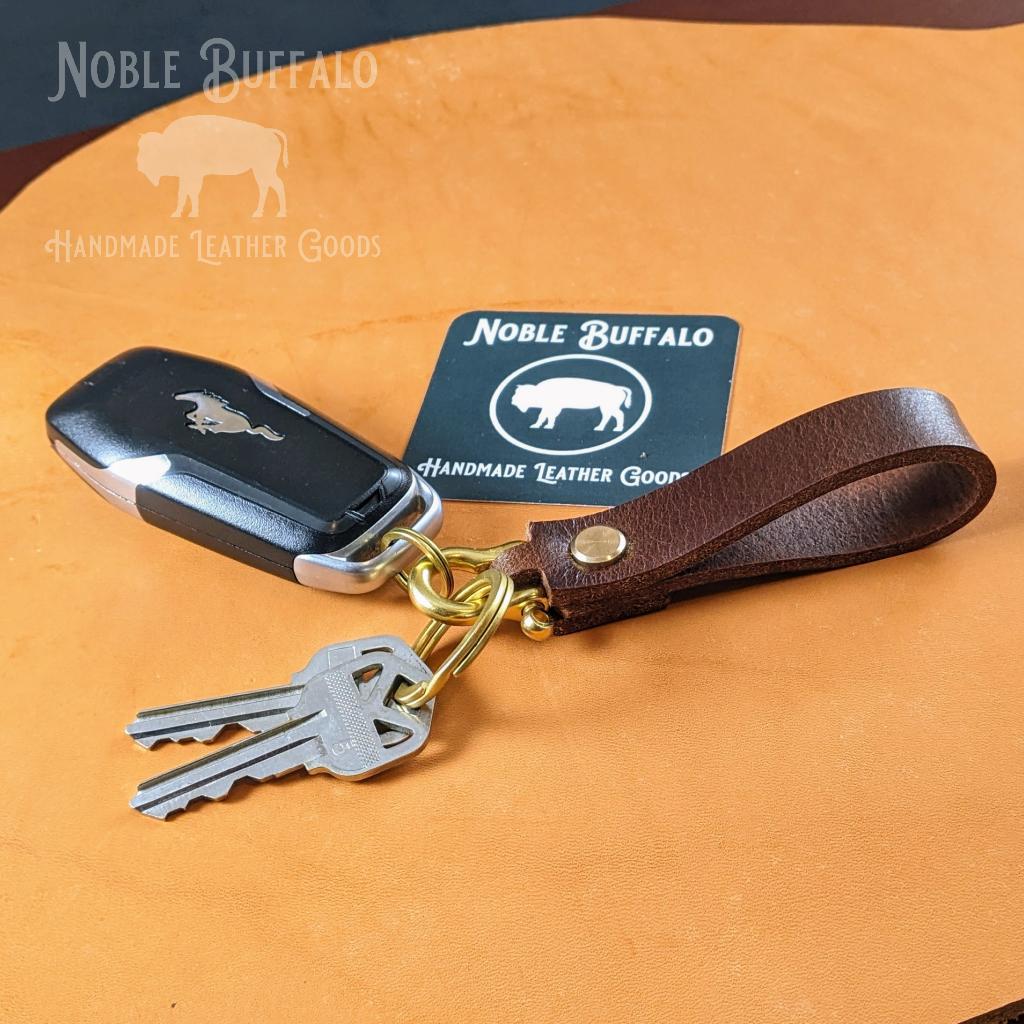This advertisement showcases a stylish keychain set against a rustic, light tan leather backdrop, emphasizing the artisanal quality of Noble Buffalo Handmade Leather Goods. The keychain features a loop of dark brown, chestnut-colored leather held together with a brass rivet and ring. Attached to the keychain are a pair of silver house keys and a sleek, black and silver key fob emblazoned with the iconic Mustang logo, indicative of a car alarm or electric ignition starter. Prominently displayed behind the keychain is a placemat or business card bearing the Noble Buffalo insignia—a white buffalo silhouette encircled, with the text "Noble Buffalo Handmade Leather Goods." This logo is repeated in a watermark-like, transparent version in the upper left corner of the image, further emphasizing the brand. The overall setup and high-quality materials highlight the craftsmanship and rugged elegance of Noble Buffalo's products.